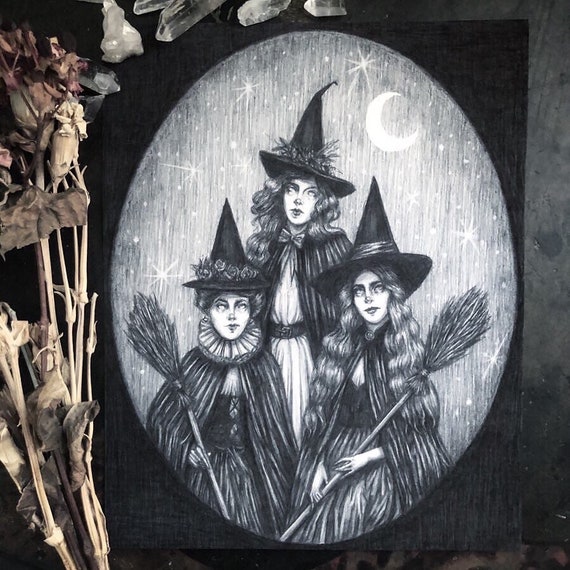This detailed pencil drawing, etched onto what appears to be a black or burnt wood surface, depicts three witches against a dark background. The witches are arranged in a subtle oval pattern with a crescent moon and numerous stars illuminating the scene behind them. All three witches sport traditional pointy black hats, each uniquely decorated: the witch on the left has flowers around her brim, the middle one has sprigs and berries, and the one on the right is adorned with a satin ribbon.

The composition shows two witches seated while one stands behind them. Both seated witches are holding brooms; the standing witch has her hair styled up, adding to her distinct appearance. The left seated witch has her hair in an updo, and the witch on the right, like the one in the middle, has long wavy hair cascading down. The expressions on their faces are serene, each smiling with closed mouths, creating a harmonious and slightly eerie atmosphere.

Additional elements enhancing the witchy, autumnal vibe include a tree branch off to the left, dried roses, and crystals positioned above the scene. These elements contribute to the overall enchanting and mystical feeling of the image, making it a perfect Halloween decoration filled with rich, intricate details.